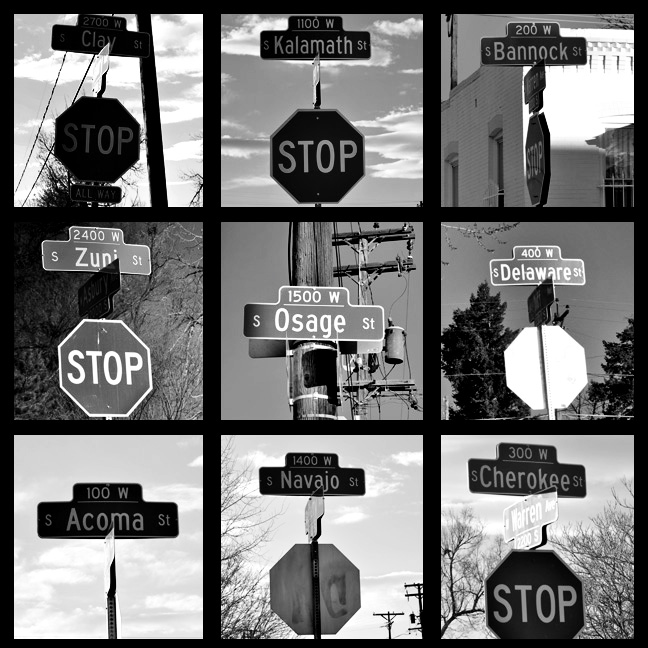The photograph is a composite of nine black and white images arranged in a three-by-three grid, each outlined in black. The central theme of the images revolves around street signs, most of which are accompanied by stop signs. 

From left to right, top to bottom, the captions on the signs read:

1. Clay - The stop sign is fully visible.
2. Kalamath Street (1100 West) - The stop sign here is also clearly seen.
3. Bannock Street (200 West) - The stop sign faces sideways and a white building is visible in the background.

Middle row:

4. South Zuni Street (2400 West) - The stop sign faces the opposite direction.
5. South Osage Street (1500 West) - The stop sign isn't visible. The background includes a telephone pole with canisters or transformers.
6. South Delaware Street (400 West) - Only the back of the stop sign is seen, likely due to sunlight.

Bottom row:

7. South Acoma Street (100 West) - No stop sign is present in this image.
8. South Navajo Street (1400 West) - The stop sign appears to face away from the viewer.
9. South Cherokee Street (300 West) - A stop sign is present, and a secondary sign pointing towards Warren Avenue is also visible.

Backgrounds in the images vary, with some showing buildings, clouds, and skies, while others include foliage and trees. The stop signs' orientations vary: some are frontal, some side-view, and one from the back.